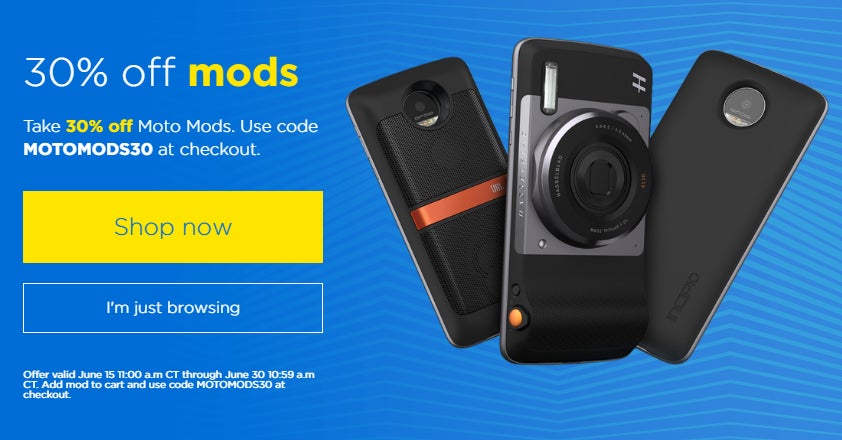**Descriptive Caption:**

Against a blue background, this advertisement showcases an enticing promotion. In the top left corner, text announces "30% off Mods," encouraging customers to "Take 30% off Moto Mod." Instructions for redeeming the discount are given, advising users to enter the code "MotoModS30" at checkout. A prominent yellow rectangle invites immediate action with the words "Shop Now," while an alternative option states, "I'm just browsing." The offer's validity period is specified, running from June 15th at 11 AM CT to June 30th at 9 AM CT.

The focal point of the ad is the display of three distinct smartphones. The first phone features a slightly rugged back with a conspicuous red bar. The second phone highlights its sophisticated camera setup, complete with a flash and what resembles a shutter button, though the camera is located on the back. The third phone stands out with its sleek silver edges and a light blue back adorned with dynamic, wavy lines, contributing to a visually engaging look. The intricate wallpaper design within the ad's background also emphasizes a motif of undulating waves, reinforcing the modern and stylish theme.